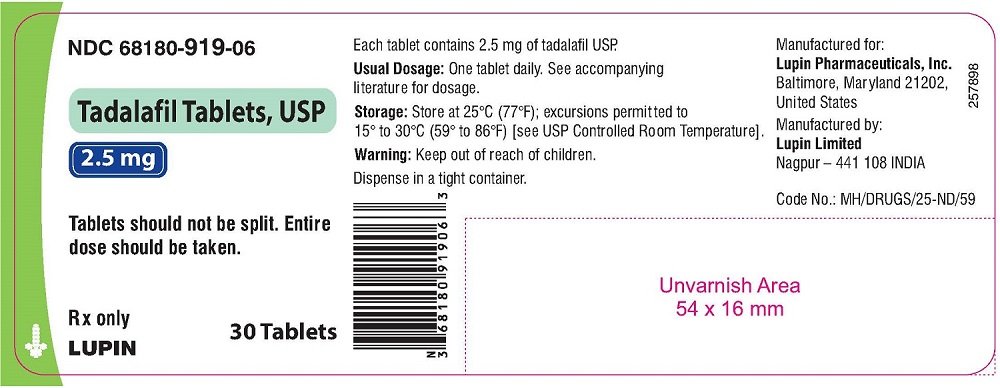This rectangular label appears to have rounded edges, with one end appearing almost pointed, likely due to a dotted outline. A green section in the corner highlights a small icon positioned at the bottom left. The label reads "NDC 6818-919-06" above bold lettering in a blue background stating "Tadalafil Tablets, USP." The dosage of "2.5 mg" is also highlighted within this blue section. Below, it advises, "Tablets should not be split. Entire dose should be taken." It is marked "Rx only" with "Lupin" and indicates that there are "30 tablets" inside.

The central part contains further information, including usual dosage guidelines, storage instructions, and safety warnings. On the right-hand side, the label lists "Manufactured for Lupin Pharmaceuticals" along with their address. There is a barcoded area below the warning section, and an unfurnished area measuring 5 by 16 millimeters is also present on the right side of the label.